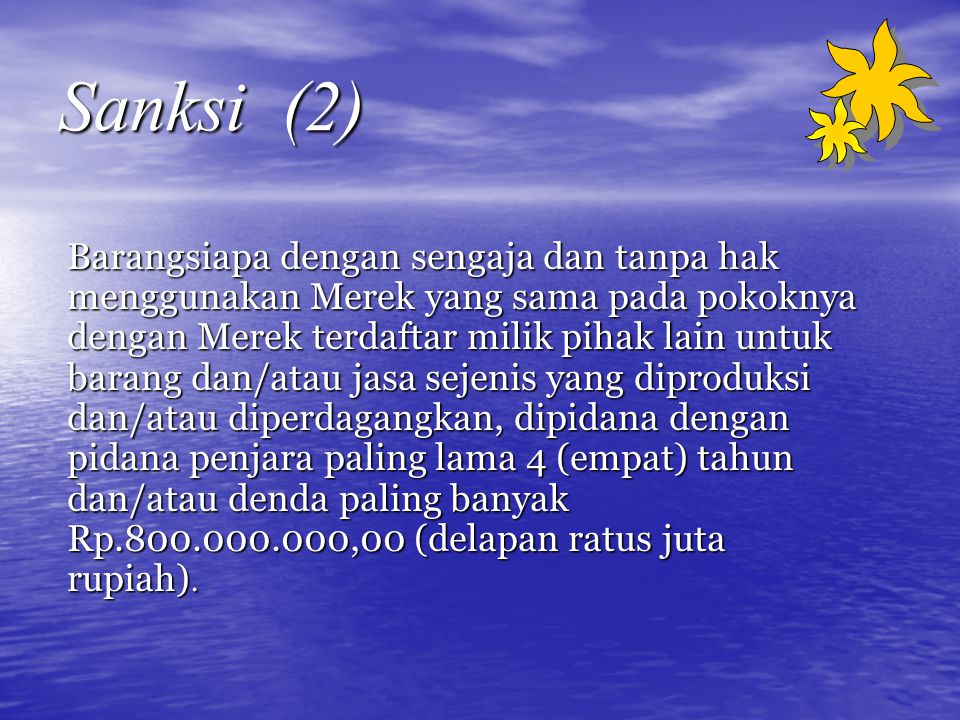The image is a detailed blend of photography, line art, and typography. It is set in a landscape orientation, dominated by a photo-realistic depiction of a bright blue ocean extending from the bottom up to the three-quarters mark of the image, reflecting light on the top left and featuring slight waves. The horizon has a light layer of white mist with barely visible land masses, topped with a sky that mirrors the ocean's blue, streaked with thin, wispy white clouds. 

In the upper left corner, there is white italic text with a black drop shadow that reads "Sanski (2)". On the opposite, upper right corner, there are two bright yellow flowers outlined in black with pale yellow drop shadows, one larger and one smaller. Below these elements, the body of the image contains nine lines of white text in an unrecognized foreign language, beginning with "BARANGSIAPA" and containing multiple spaces and slashes between the words. The entire visual composition gives the impression of a computer screen displaying a definition or informational text across a serene seascape background.